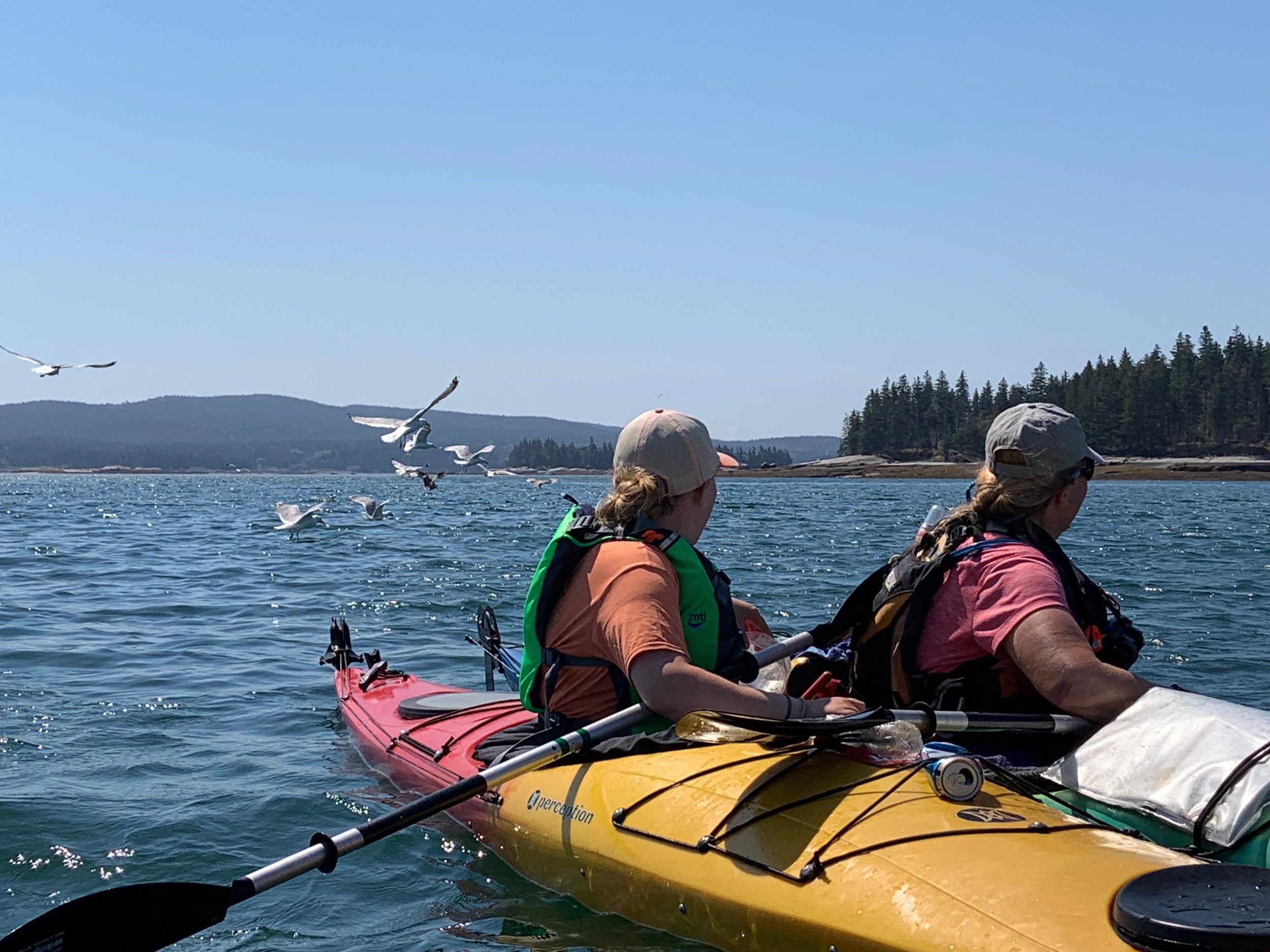In this captivating outdoor scene, a photograph captures two slightly overweight women kayaking on a tranquil, blue lake. They are paddling together in a tandem kayak, which is vibrant yellow at the front and fades into a pinkish-red at the back. Each woman, indistinguishably facing away from the camera, wears a baseball cap and a life vest over their t-shirts—a pinkish-red shirt on one and an orange shirt on the other. The word "Perception" is visible on their kayak, indicating its brand. One of their oars is visible extending towards the left side of the image. The women appear to be looking back at a flock of large white birds, likely seagulls, that are either flying or landing on the water behind them. The serene lake is encircled by a picturesque backdrop of low hills and distant mountains adorned with lush, dark green pine trees, suggesting a setting that could be somewhere in the Pacific Northwest. The scene is bathed in the clear blue sky of a perfect day, adding to the peaceful and enchanting atmosphere of the moment.